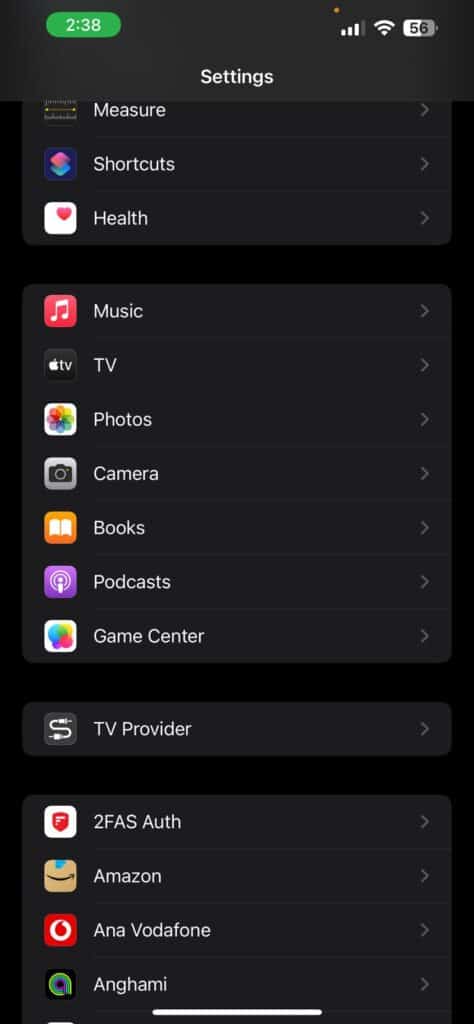This is a screenshot of a settings screen on an unknown Android device. The top of the screen displays the time as 2:38 within a green capsule, along with three to four bars of cellular signal, a full Wi-Fi signal, and a battery at 56% capacity. The settings screen features a dark background and is partially scrolled down to reveal some options labeled "Measure," "Shortcuts," and "Health," each with right-facing arrows indicating they can be tapped for more details or toggles.

Beneath these options is a panel with seven icons:
1. A red note, likely for a music app.
2. An Apple TV icon, signifying the TV app.
3. An icon resembling a rainbow ring, probably for the Photos app.
4. A camera icon for the Camera app.
5. An open book, representing the Books app.
6. A small eye with radiating lines, indicating the Podcasts app.
7. A cluster of bubbles, denoting the Game Center app.

Further down, there is another gray line labeled "TV Provider" with an associated cable link icon shaped like an 'S'. Below this section is an area titled "2FAS Authorization" featuring a badge icon. Additional icons within this area include:
1. A smile in a box with "Amazon" to the right.
2. A twisted red teardrop within a white circle and a blue square, possibly indicating a Vodafone service.
3. A multicolored "A" logo labeled "NGAMI," spelled N-G-A-M-I.